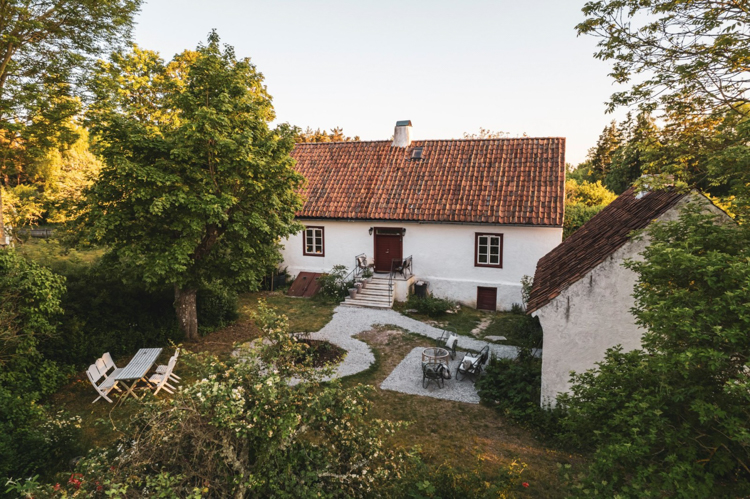This outdoor scene depicts a charming, white, cottage-style home with a terracotta roof accented by black and a central white chimney. The front of the house features a dark brown door framed by two windows with brown borders, each consisting of six separate glass panes. Access to the door is provided by a white staircase with five or six steps and a black wrought iron railing. To the left of the stairs is a storm cellar with two brown doors, and in front of the steps lies a circular gravel pathway, with one part leading straight ahead to a gravel area featuring a flower bed in its center.

To the right of the main house, there is another white structure, possibly a guest house or a garage, with a gravel path connecting both buildings. This secondary building closely resembles the main house and adds to the rustic charm. The yard is equipped with ample seating areas, including a large table with six chairs, a white picnic table, and a round fire pit without adjacent seating. Surrounding the entire property are large trees, shrubs, and dense foliage, providing a serene and secluded atmosphere.